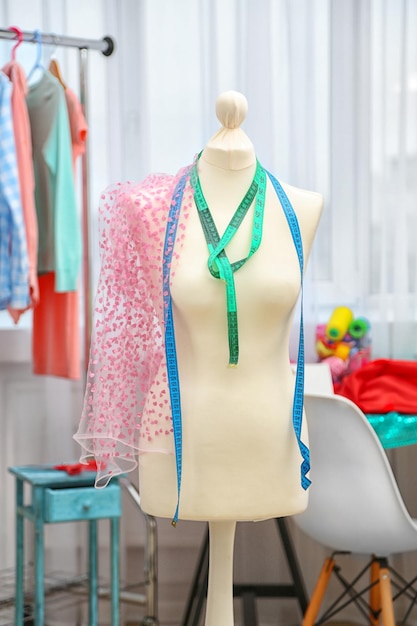The image depicts a detailed scene likely from a seamstress's workspace, featuring a headless and legless female-shaped mannequin prominently in the center. The mannequin is adorned with two measuring tapes, one blue and one seafoam green, draped around its neck and shoulders. Over its right shoulder, a sheer, translucent garment dotted with pink, flower-like shapes hangs elegantly. In the background, gauzy white curtains obscure a potential city view, blending seamlessly into the setting. To the mannequin’s left stands a metallic garment rack holding various shirts—pink, teal, peach, and blue checkered. Below this rack, a compact teal table with a slightly open drawer, has a pair of red scissors resting on top. On the right side of the frame, there is a white, modern-looking chair with brown legs, pulled up to a table adorned with miscellaneous sewing tools and materials, covered by a blue tablecloth. The overall arrangement and elements suggest a creative environment dedicated to clothing design and tailoring.